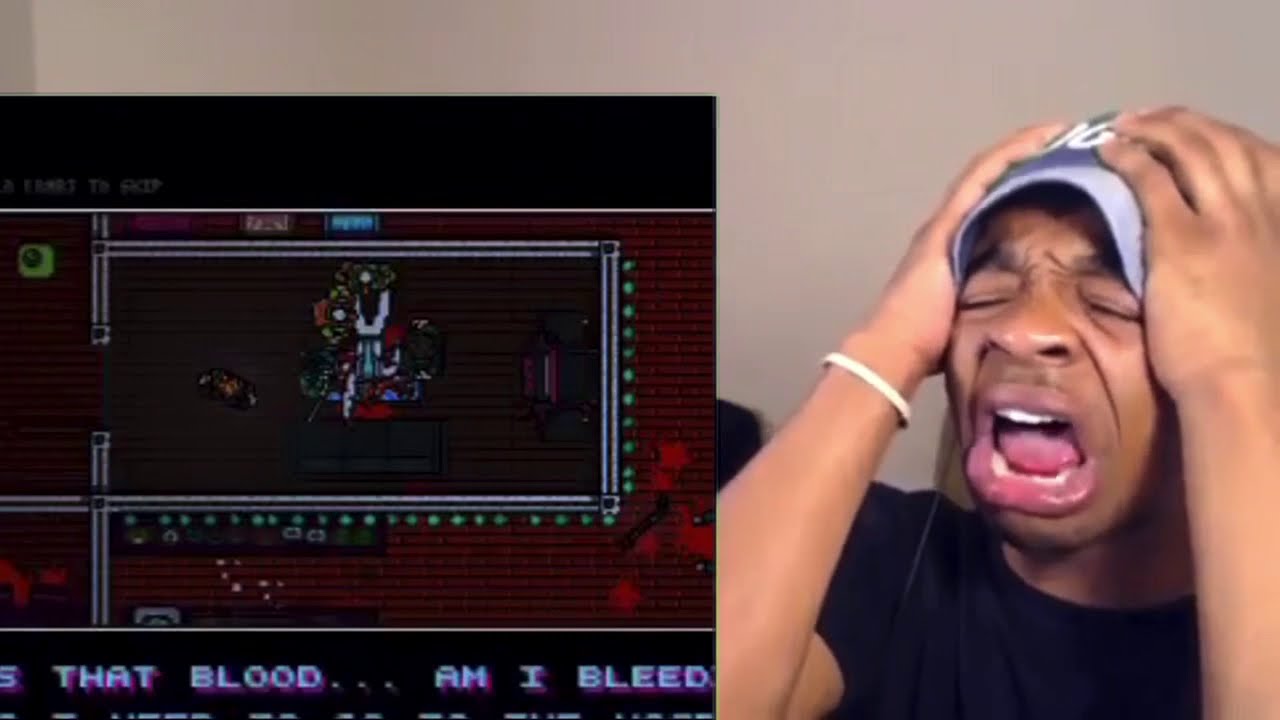The image features an anguished black man, his mouth wide open in a scream, possibly due to a game loss. His eyes are tightly shut, and he's holding his blue ball cap with both hands on top of his head. He's dressed in a black t-shirt, revealing the form of one arm and most of the other, and he's wearing a silver or white bracelet on his right wrist. Behind him, there's a light or dark tan wall. To the left of the man, there is a screenshot that appears to be from an old-style video game, with dark visuals. The text at the bottom of the screenshot reads, "that blood... am I bleed," partially obscured and in blue lettering. The game graphic seems to depict a person in long robes standing on a basketball court-like design, surrounded by a red section resembling a rug with an indistinct dark red object within it.